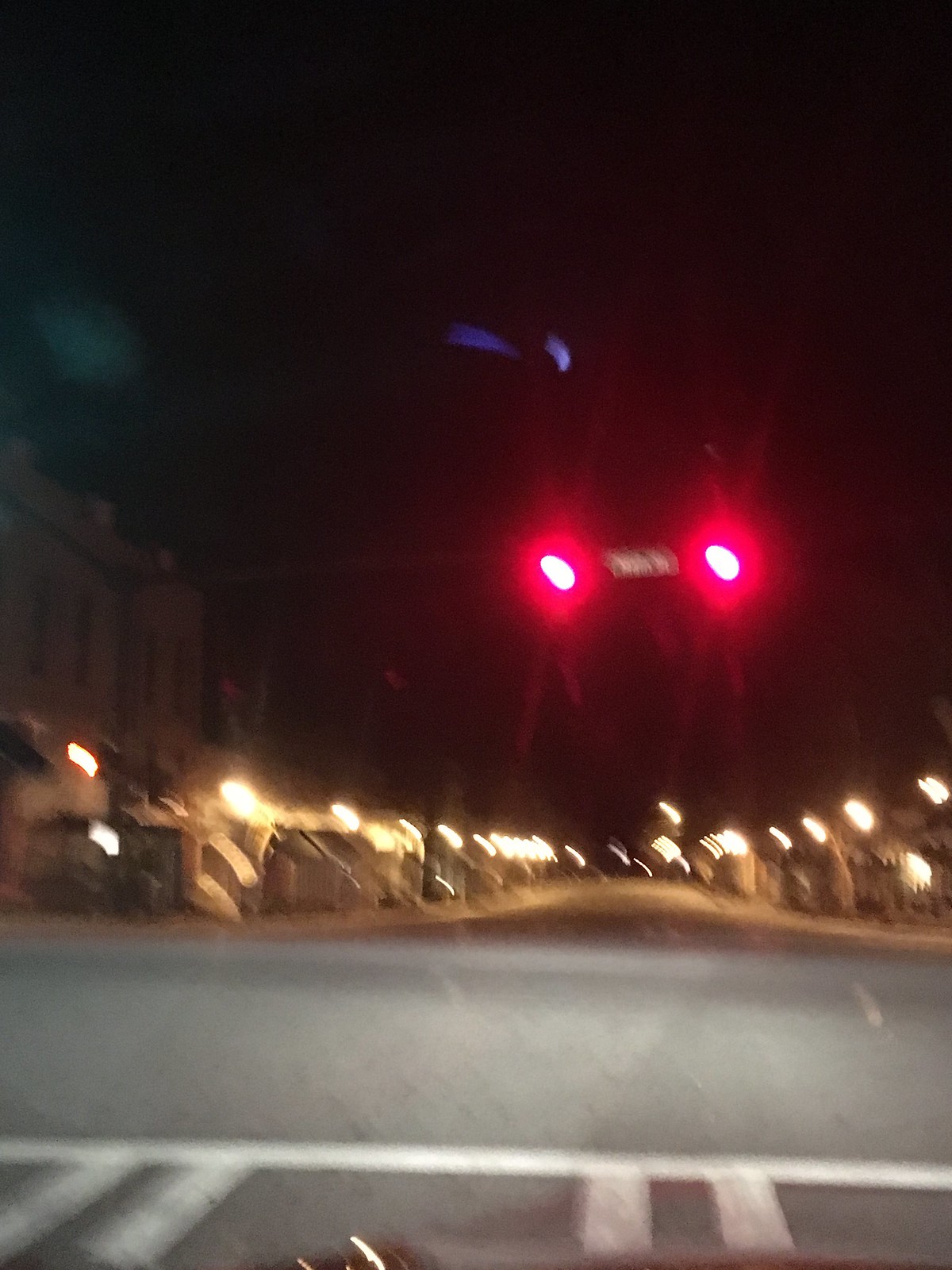The image depicts a blurry nighttime scene as seen from the passenger side of a car. The primary focus is on two glaring red traffic lights ahead on what appears to be an almost empty street. Between these lights is a small street sign, which under close inspection seems to read "Main Street" in white letters against a green background, typical of standard street signage. The scene is illuminated by multiple yellow street lights, casting a yellowish hue across the street, with the sky pitch black overhead. In the foreground, the subtle outline of a car's front and an illuminated crosswalk with white stripes can be discerned. The road itself is gray and flanked by an array of white lights from buildings or stores, stretching into the distance. The overall image is out of focus, suggesting movement or an unsteady hand while capturing the shot.